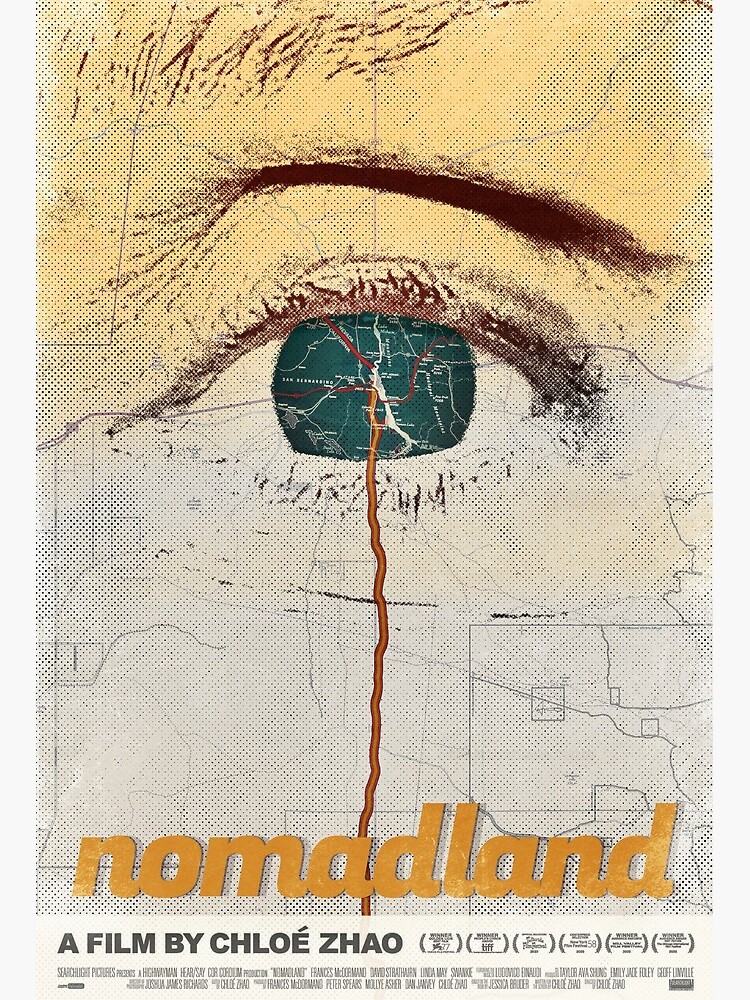This is a detailed movie poster for "Nomadland," designed to resemble a hand-drawn map. The upper portion of the poster features a peach or flesh-toned background with a brown section resembling an eyebrow, giving the impression of the upper edge of an eye. The center of the image showcases a round green area, colored to look like an eyeball, with an orange river-like line running downward, evoking a map-like journey. The lower half transitions to a white background and includes intricate map details. In large orange letters, the title "Nomadland" is prominently displayed at the bottom. Beneath this, in smaller black text, the poster credits "a film by Chloe Zhao." Further down, in even smaller and less readable text, is the standard information listing important contributors and studio logos.